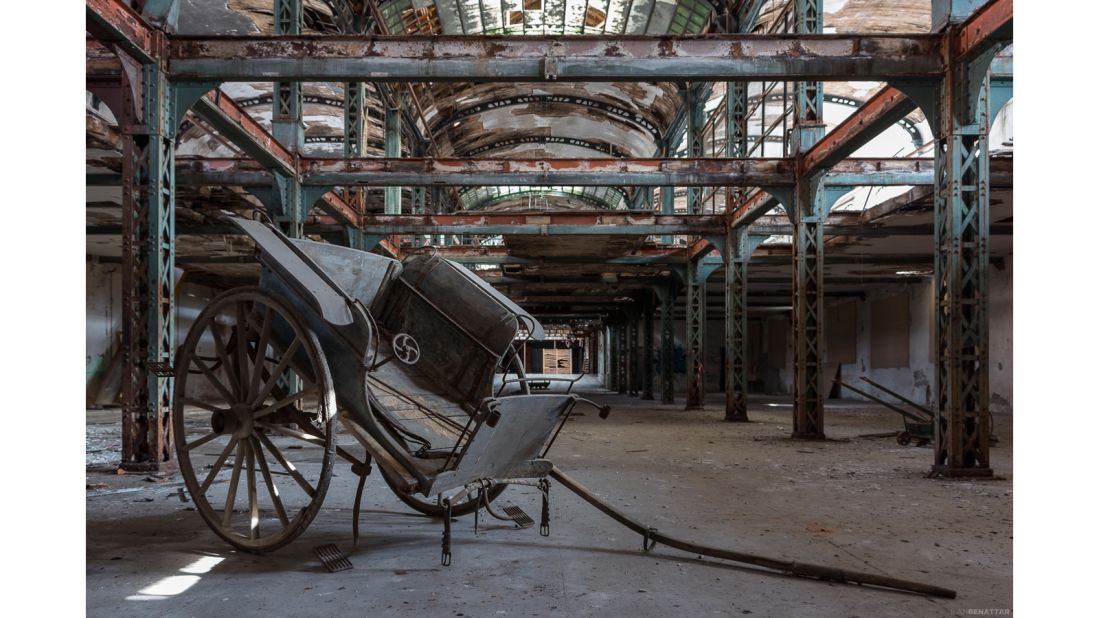The image depicts the interior of an old, abandoned warehouse with a weathered, exposed structure. The building's skeletal frame is composed of green steel beams, now heavily rusted to shades of brown and grey. The ceiling features glass windows that allow daylight to stream in, illuminating the neglected, dusty concrete floor below. The warehouse is spacious, with beams running along the left and right sides and across the top, creating an open, industrial atmosphere. On the second floor, partially visible, are additional floor areas. In the foreground, positioned towards the left side of the image, is a vintage, hand-driven cart—a relic from a bygone era. This cart, black and grey in color, features large wheels, a sitting platform with raised armrests, back support, pedals, chains, and a pulling rope, leaning slightly due to its detached state. The overall setting is one of decay and abandonment, capturing a sense of history and erosion.